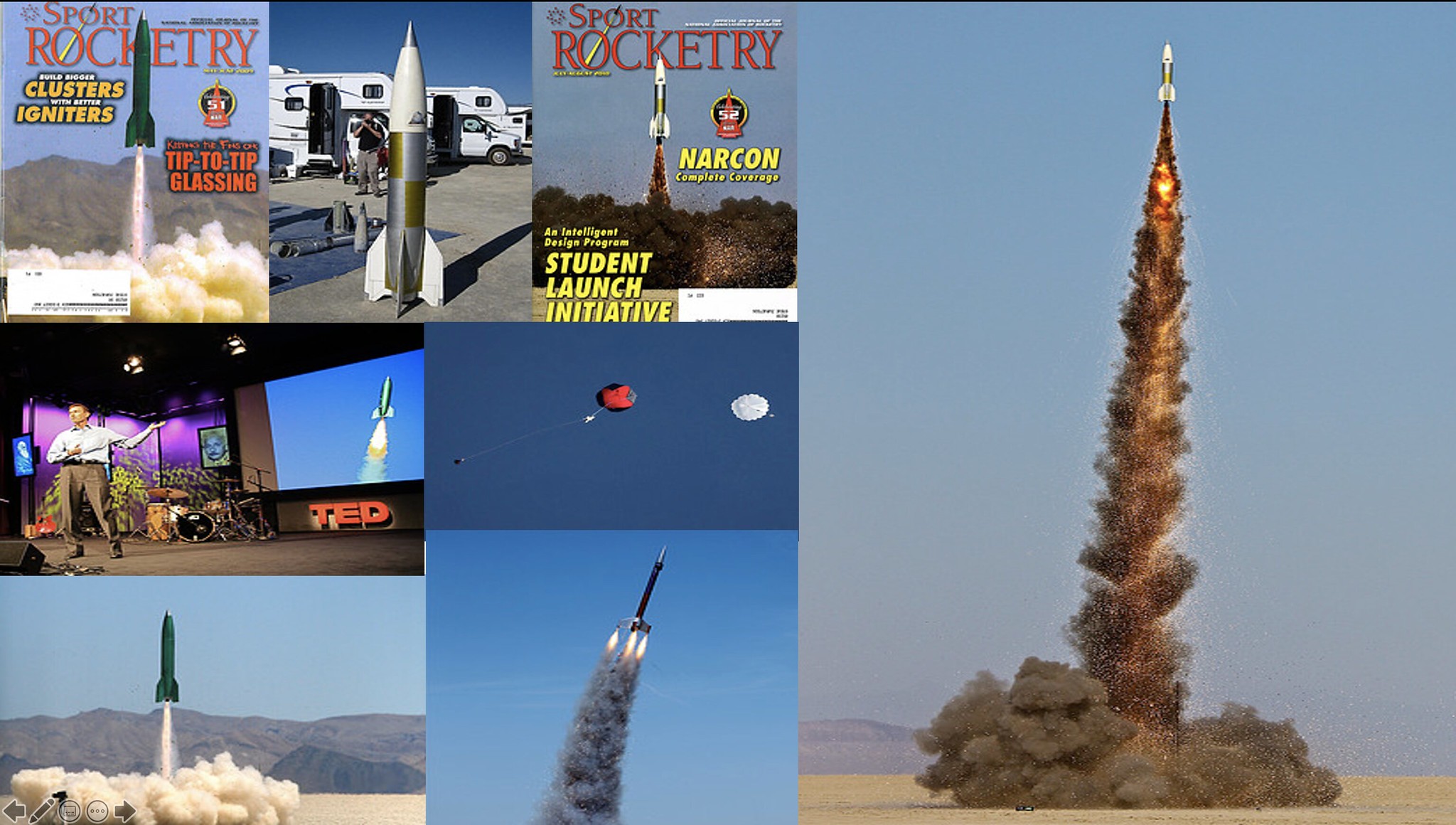The image is a detailed horizontal collage consisting of about eight different photographs related to sport rocketry, seamlessly merged together. Dominating the right half is a striking image of a large white-and-black rocket launching skyward, trailing flames and a thick plume of grayish-brown smoke against a clear blue sky. The left half of the collage is rich with varied scenes: at the top left are two covers of "Sport Rocketry" magazine, each showcasing rockets in mid-launch with bold red lettering. Below these, a prominent foreground image displays a sizable rocket on the ground in front of several RVs, with a man in gray pants and a black short-sleeved shirt photographing it. Adjacent is an action shot of a vibrant green rocket ascending, smoke billowing beneath it, set against a hilly backdrop. Further down, another rocket takes flight, its triple flame and smoke trail vividly depicted as it angles to the right. To the right of this is a TED talk scene, where a speaker stands before a screen displaying a rocket mid-launch. Lastly, an image of a parachute—possibly from a descending rocket—adds to the diversity of rocketry activities represented. The clear blue skies and bright sunshine provide a cohesive and vivid backdrop across all scenes, tying the energetic montage together into a comprehensive advertisement for sport rocketry.